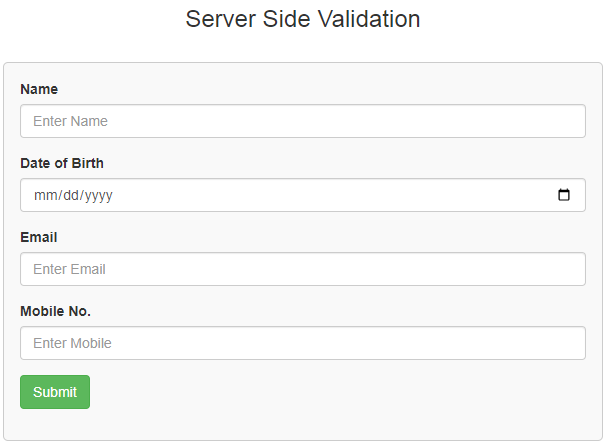**Screenshot Description: Simple and Clean Form Design**

The screenshot captures a simplistic and clean user interface dedicated to server-side validation. Dominating the top of the image is the phrase "Server-Side Validation" displayed prominently. Below this header lies a rectangular input area bordered by a thin gray line with elegantly curved corners.

The form consists of four labeled entry fields, each preceded by a bold black header: 

1. **Name:** Accompanied by an entry field placeholder that says "Enter Name."
2. **Date of Birth:** With an entry field formatted as "mm/dd/yyyy" and a small calendar icon to the right for selecting a date via a dropdown calendar interface.
3. **Email:** Featuring an input field with the placeholder text "Enter Email."
4. **Mobile Number:** Containing a field labeled "Enter Mobile."

Each entry field is highlighted in gray, maintaining coherence with the form's minimalist aesthetic.

On the bottom left of the form lies the "Submit" button, characterized by its green background, white text, and rounded corners, adding a touch of softness to the overall design.

Enveloping this neat arrangement is a pristine white background devoid of any extraneous details, such as drop shadows or additional graphics, which ensures the layout remains uncluttered and straightforward.

Overall, the image showcases a well-organized, user-friendly form section of an unidentified application or website. The design's emphasis on simplicity and clarity makes it a standard and efficient layout for user data entry.